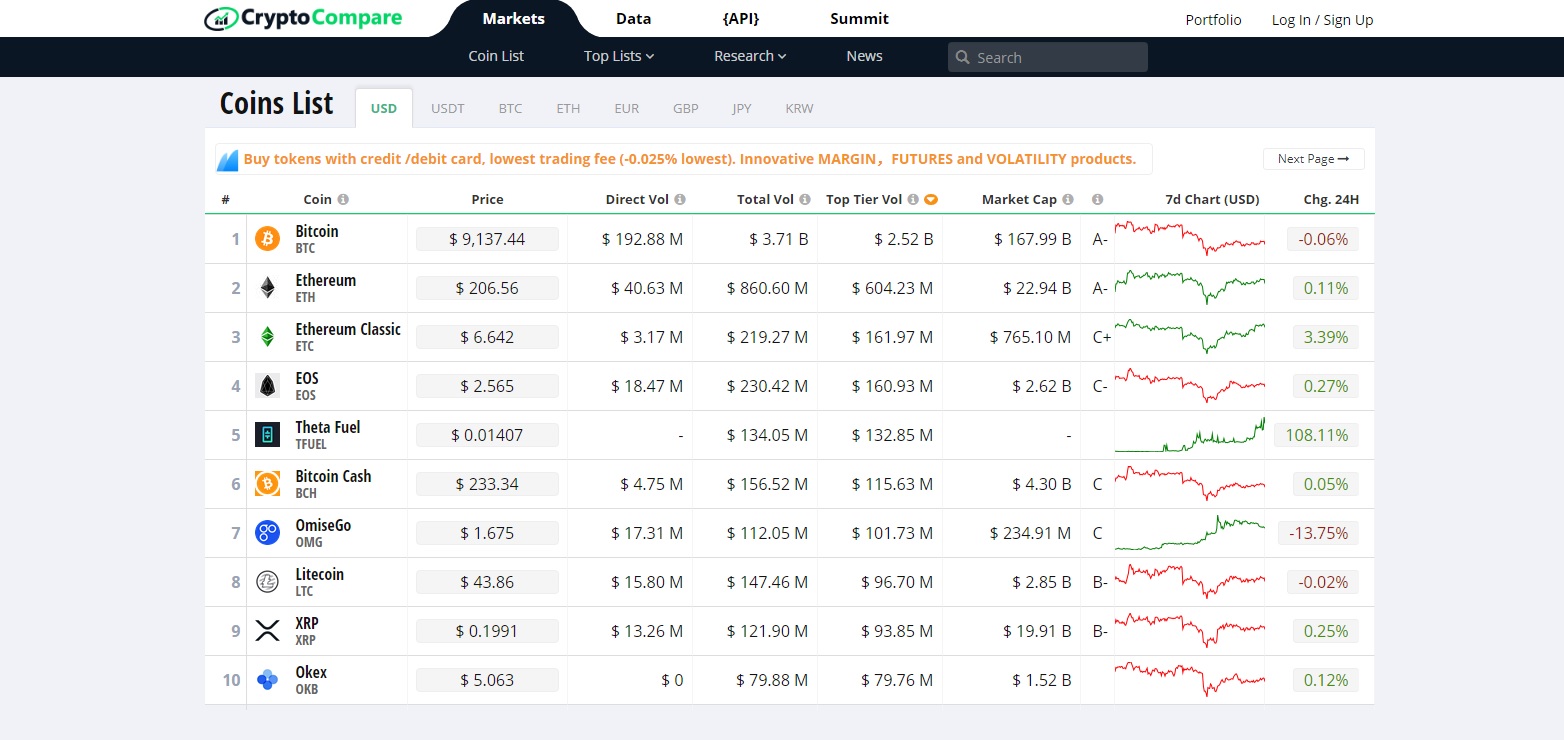Here is a cleaned-up and detailed caption for the described image:

---

The screenshot showcases the user interface of a desktop application named "Crypto Compare." The interface's top-left corner prominently features the application's name. The active tab highlighted is the "Markets" tab, situated alongside other primary navigation tabs including "Data," "API," and "Summit." Further to the right, slightly separated, are the "Portfolio" tab and options for "Login" or "Signup."

Directly below the "Markets" tab resides a secondary navigation bar featuring options such as "Coin List," "Top Lists," "Research," "News," and a "Search Bar." 

The main section of the interface displays a list of various cryptocurrencies with the currencies supported being USD, USDT, BTC, Ethereum, EUR, GBP, JPY, and KRW (with a possible mix-up, as KRW is South Korean Won, not Polish Zloty). Below the list of currencies, there are promotional messages including "Buy Tokens with Credit, Debit Card," "Lowest Trading Fee at -0.025%," "Innovative Margin," "Futures," and "Volatility Products."

Further down, the detailed table layout showcases several columns: coin, price, direct volume, total volume, top-tier volume, market cap, 7-day chart, values in US dollars, and percent changes within the last 24 hours.

The top ten listed cryptocurrencies are:
1. Bitcoin (BTC)
2. Ethereum (ETH)
3. Ethereum Classic (ETC)
4. EOS (EOS)
5. ThetaFuel (TFUEL)
6. Bitcoin Cash (BCH)
7. OmiseGO (OMG)
8. Litecoin (LTC)
9. XRP (XRP)
10. OKEX (OKB)

---

This caption provides a comprehensive and organized description of the image, detailing the content and layout of the application interface.